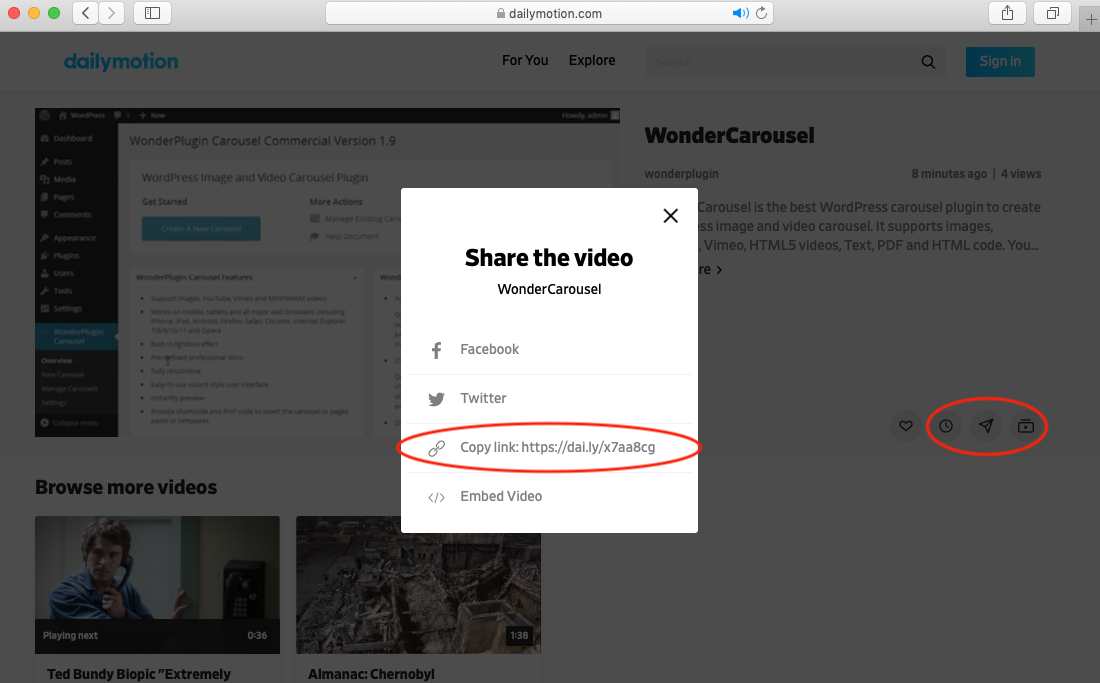The image showcases a webpage from DailyMotion, viewed on a web browser. At the very top, the URL bar displays "dailymotion.com" accompanied by a secure lock icon, all in black. Adjacent to this, a notification bell, a volume control icon highlighted in blue, and additional interface buttons are visible, including a square with an upward arrow, two overlapping squares, and a gray box with a plus sign.

On the browser's left side, there are red, yellow, and green dots typically associated with window controls, followed by arrows pointing left and right, and a square-within-a-square icon. The webpage background is muted gray, with "Daily Motion" branded in blue at the top left corner.

Prominently displayed in the center are tabs labeled "For You" and "Explore." At the top-right, a blue sign-in button with white text is noticeable. Along the left side of the page sits a black vertical sidebar listing multiple categories, partially obscured by a white pop-up.

This pop-up, titled "Wonder Plugs, Carousel Features," outlines eight features in a blurred text, interrupting the underlying content. Above, a banner reading "Share the Video" precedes sharing options for Facebook, Twitter, and a link, which is highlighted in red as "https://dai.ly.x7aah8cg". An embed video option is also displayed beneath this.

To the left of the pop-up, the main page includes a section labeled "Browse More Videos," previewing two video thumbnails. The first shows a man on a phone, labeled "Playing Next 0.36 seconds," while the second appears unclear but is tagged "1 minute 38 seconds" with the title "Almanac Chernobyl." Additional visible text mentions a video about Ted Bundy.